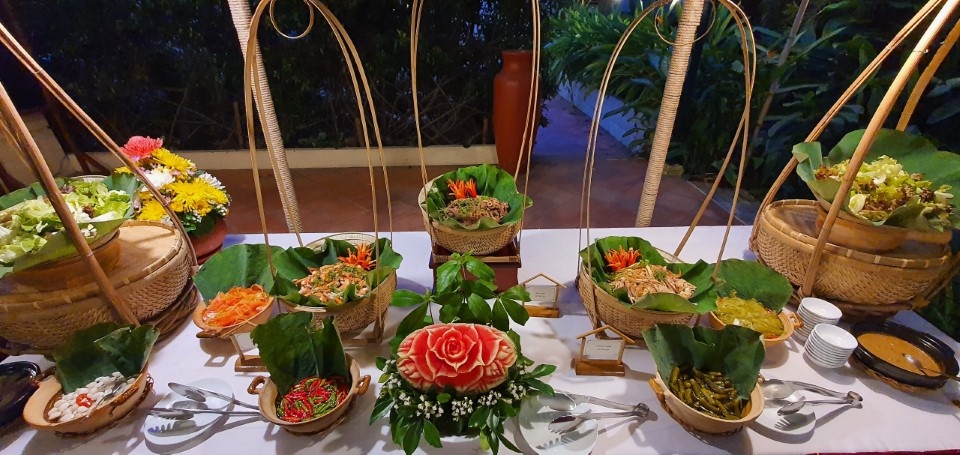The image presents a vivid and meticulously arranged dinner buffet set on a white tablecloth, possibly located in an outdoor courtyard adorned with lush greenery. At the heart of the table, a striking orange flower serves as the centerpiece, complemented by additional colorful blooms including pink and white roses. Surrounding the centerpiece, various dishes are artfully displayed on a wooden platform. Notably, the spread includes a mix of salads—carrot, garden, bean, and Mexican—along with other items that resemble fresh vegetables and flowers, perhaps even small bowls of soup, all garnished with lettuce leaves. Intriguingly, there are no plates, just utensils for handling the food. The setup includes around ten dishes, with several seeming to be larger, main courses. The arrangement also features clamps on both sides for serving, and an orange vase sits in the background, hinting at a possible Mexican culinary theme with elements like peppers, tortillas, salsa, and chips present among the dishes.